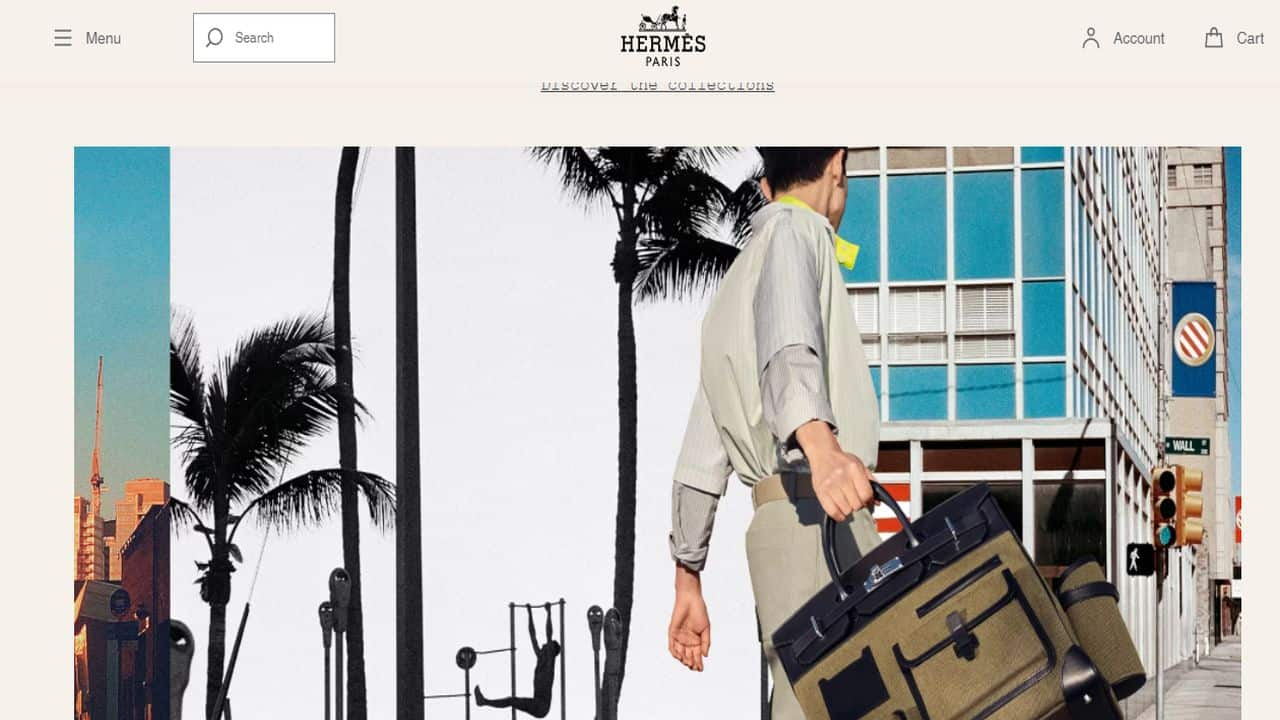This is a screenshot from the Hermes Paris website, set on a pale lavender background, showcasing the website's top navigation bar and a promotional image. 

At the top left corner of the page, there is a "Menu" option denoted by three horizontal lines. Adjacent to the "Menu," a white search bar is provided for easy navigation. Centrally positioned is the company name, "Hermes Paris," with their iconic logo placed above it. To the right side of the navigation bar, there is an "Account" button with a small person icon, followed by a "Cart" button.

Below the navigation bar, the main image features a scene from a sunny afternoon in a city. The photograph captures a white man with short brown hair, who is about to cross a street. He is carrying a light brown leather Hermes tote bag with dark brown or black leather detailing, which swings by his right side as he walks. The man, facing away from the camera, appears to be approaching a crosswalk where a "WALK" signal is illuminated, and a green light indicates it is safe to proceed. The street he is on is named "Wall."

In the background, there are palm trees, parking meters, and the silhouette of someone performing a gymnastic routine on uneven bars. The sky is a vibrant blue, adding to the bright and lively atmosphere. Across the street stands a multiple-story building adorned with turquoise blue panels, adding a modern architectural touch to the scene.